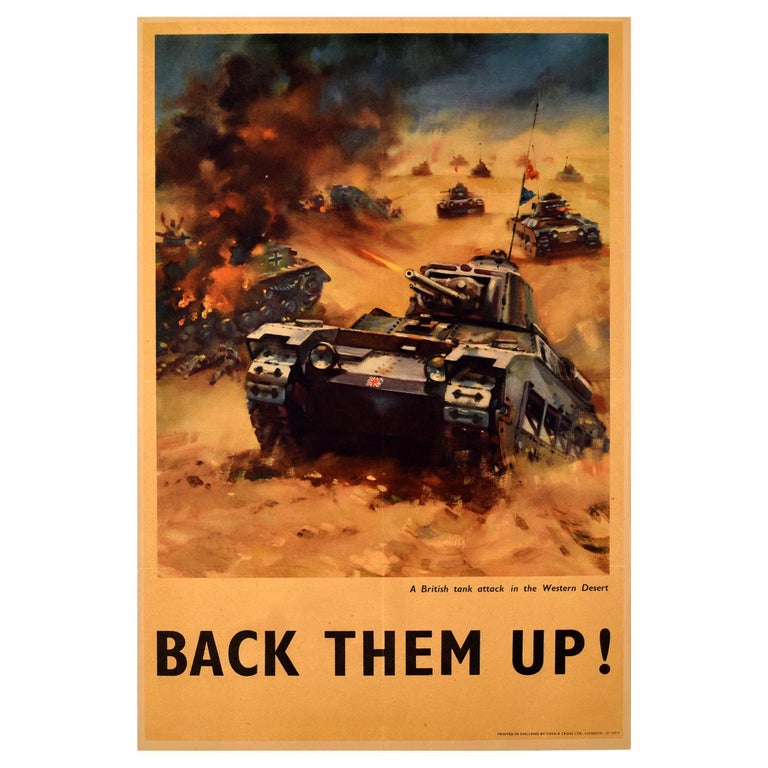The image is a vintage war propaganda poster, featuring an intense battle scene with a dozen or so tanks engaged in combat on a sprawling, open dirt field in what looks like the Western Desert, possibly Northern Africa. The background is tinted with a tannish color, filled with billowing smoke and the chaos of warfare. Several tanks are damaged or on fire, while others actively fire their cannons, with one prominently shooting an orange streak of fire. A lone tank can be seen climbing a desert hill, adding to the dynamic composition. The ground beneath the tanks carries an orange undertone, reminiscent of hay. The poster prominently displays the slogan "BACK THEM UP!" at the bottom in large, bold letters, with a smaller caption beneath it that reads, "British tank attack in the Western Desert."